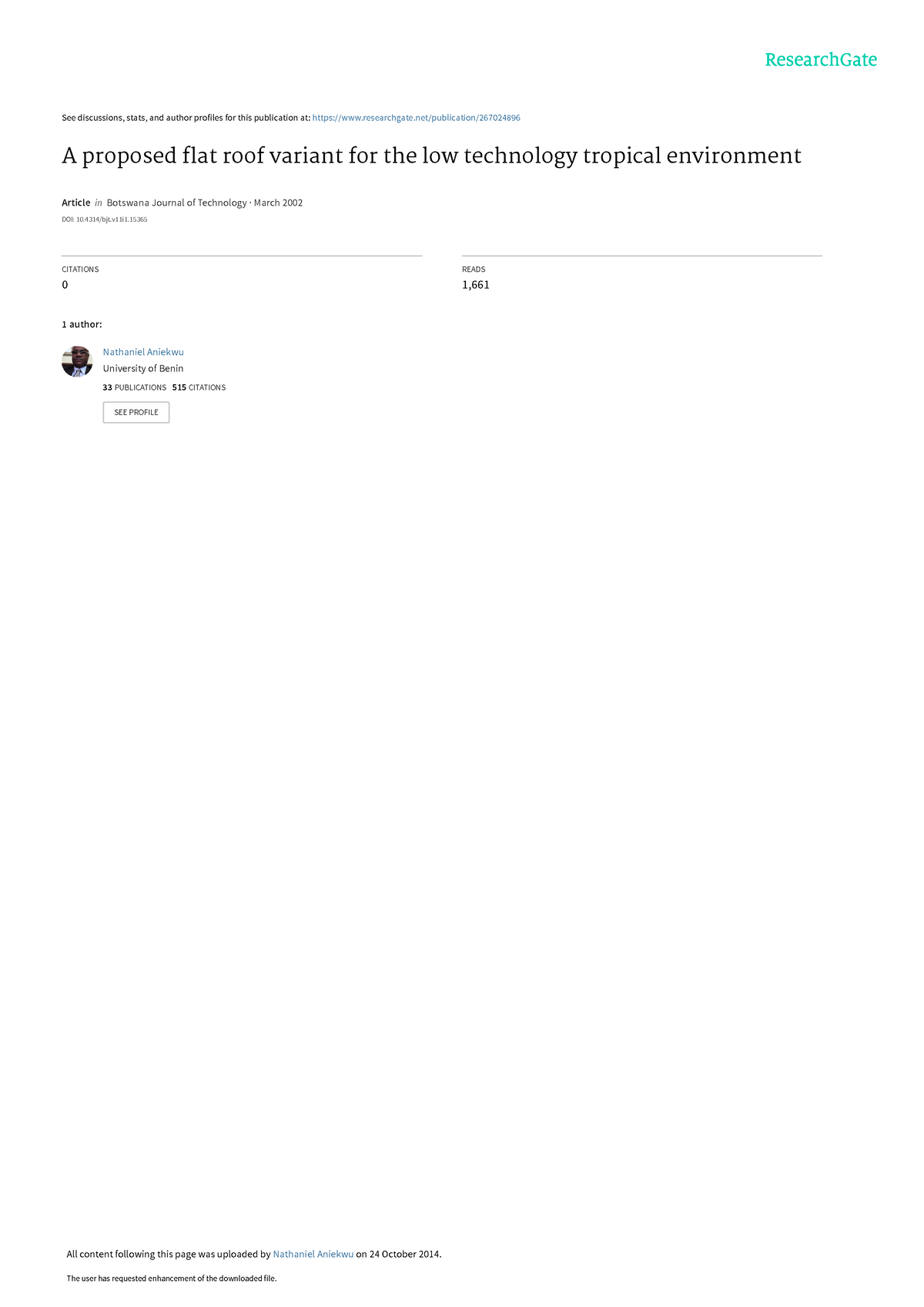This is a screenshot of a web page, specifically from ResearchGate. In the upper right corner, highlighted in green text, is the brand name "ResearchGate." On the left side at the top is a description and link indicating the website's nature, although the text is too small to decipher clearly. 

The main title of the web page reads "A Proposed Flat Roof Variant for the Low Technology Tropical Environment." Beneath this title, in very small text, it mentions "Altschreis and Botswana Journal of Technology, March 2002." Directly below this, there is an icon representing the author, accompanied by the name "University of Berlin." It indicates that the author has published 13 publications and created 813 works.

To the right of the author's information, there is a button labeled "See Profile." At the very bottom of the page, a note mentions that all content was last updated on October 24, 2014, with a faint link included in this statement.